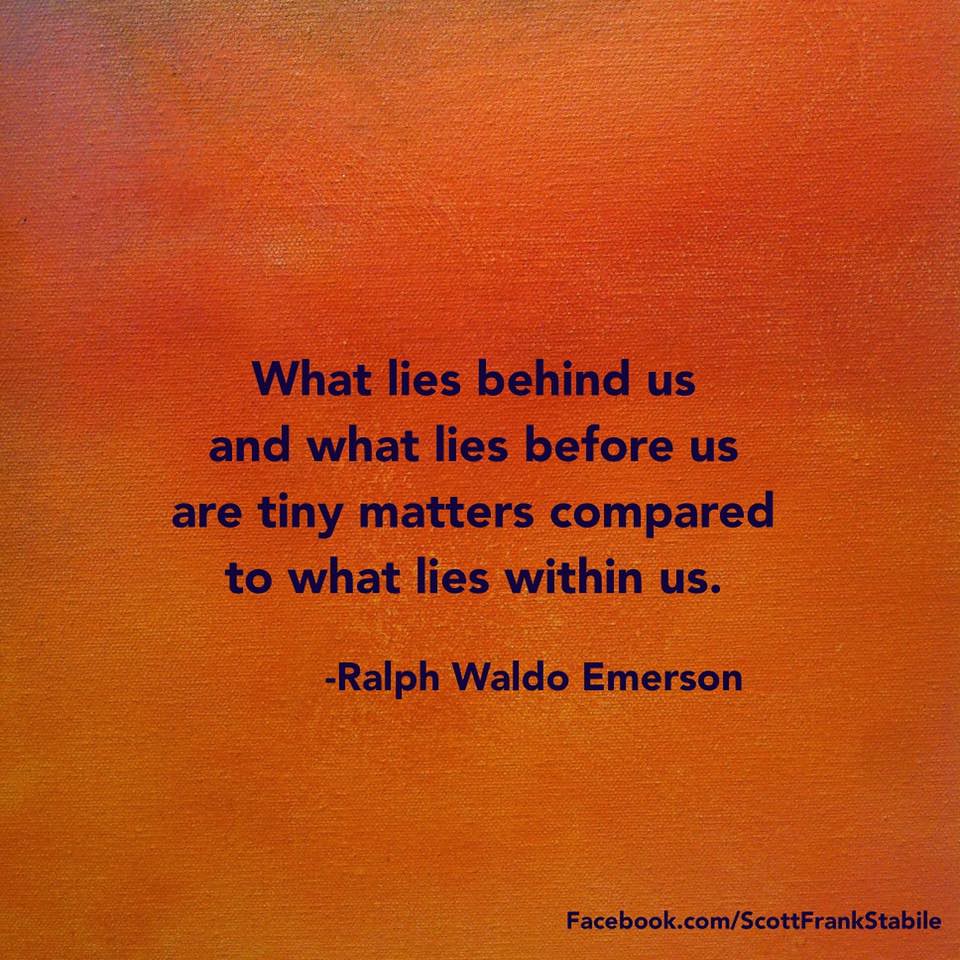The image is a square graphic designed as either an inspirational poster or a PowerPoint slide. The background is a textured, painted canvas with various shades of sunset-like orange, ranging from light orange to a darker red. In the center of the image, superimposed in large dark blue font, is a motivational quote by Ralph Waldo Emerson: "What lies behind us and what lies before us are tiny matters compared to what lies within us." Directly below the quote, in slightly smaller font, is the attribution to Ralph Waldo Emerson. In the bottom right-hand corner, a URL is displayed in the same dark blue font: "facebook.com/ScottFrankStabile," with no spaces. The textured look of the background suggests that it might be a photograph of the quote printed on an actual canvas.